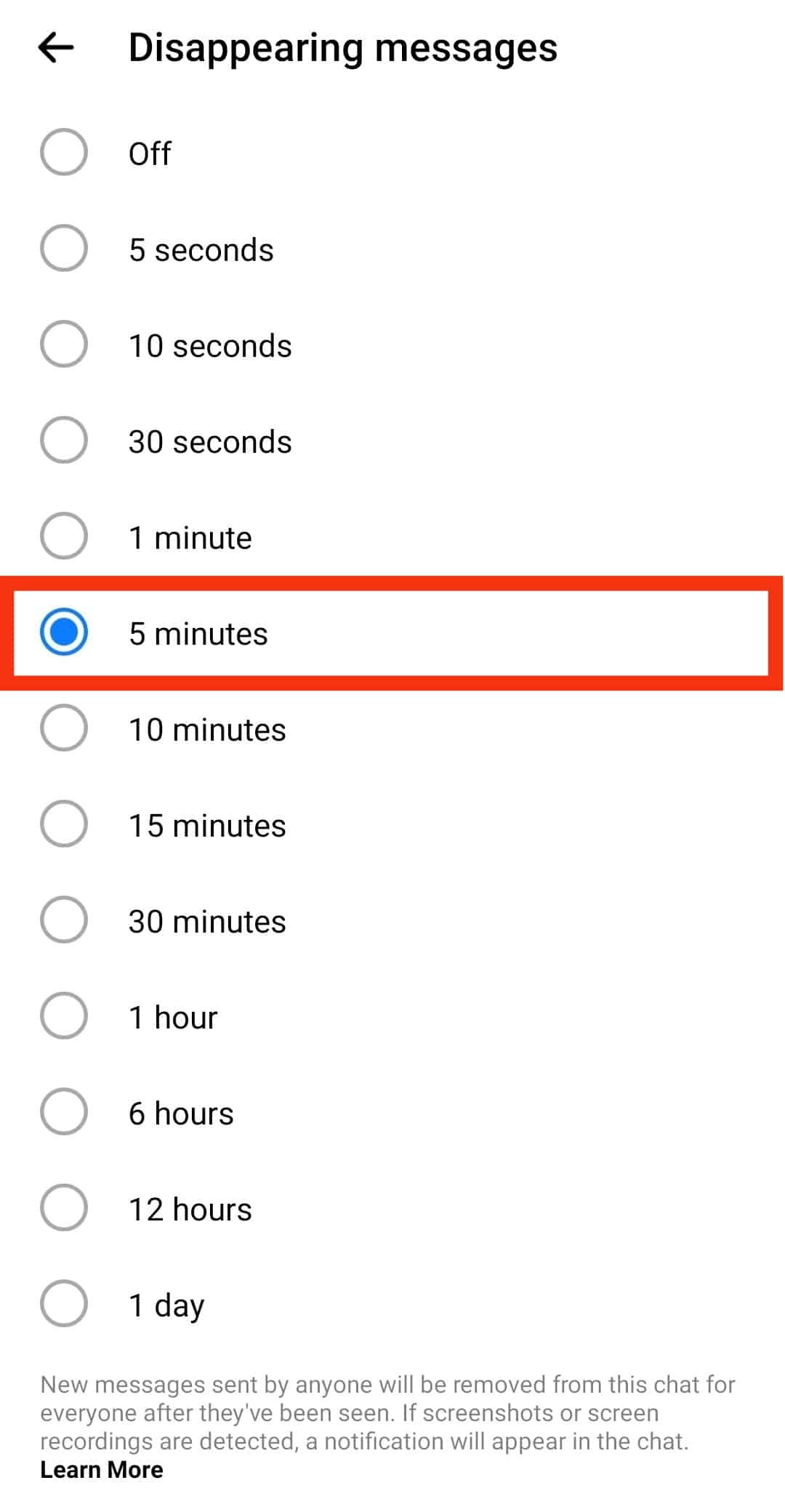The vertical image appears to be a screenshot from a computer or phone interface where users can select the duration for which messages will be visible before disappearing. The background is plain white, emphasizing the options laid out on the screen.

At the top, a bold arrow points to the left next to the bold text "Disappearing Messages". Below this header, there is a list of options represented by unfilled circles with gray outlines, set against the white background. Each option is labeled in a light black or gray font. The options available are: Off, 5 seconds, 10 seconds, 30 seconds, 1 minute, 5 minutes, 10 minutes, 15 minutes, 30 minutes, 1 hour, 6 hours, 12 hours, or 1 day.

The "5 minutes" option is selected, indicated by a blue filled circle and a thick red rectangular box around it. At the bottom of the image, there is informative text stating: "New messages sent by anyone will be removed from this chat for everyone after they've been seen. If screenshots or screen recordings are detected, a notification will appear in the chat", followed by the bold directive "Learn more".